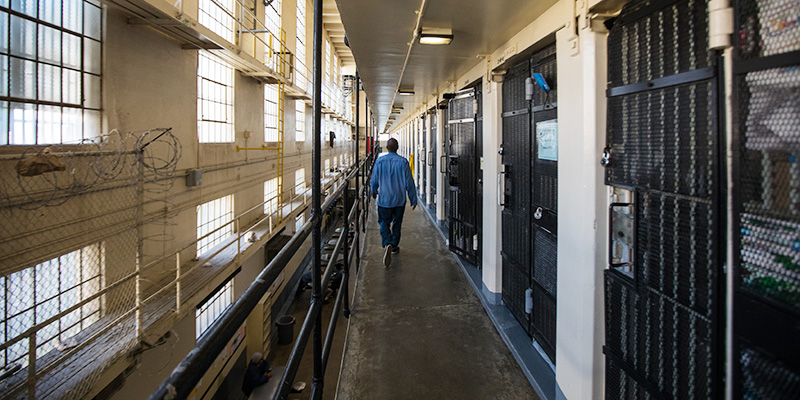The scene depicts the interior of a multi-level prison walkway. The viewer is positioned on an upper floor, which has a heavy-duty, black metal mesh cage lining the right-hand side with a long row of secured cell doors. The floor is a solid concrete slab with a black handrail running along the left side. A man, dressed in a blue long-sleeved shirt, black jeans, and tennis shoes, is walking along this path. The left side features walls covered in windows, some of which are heavily gated with barbed wire, allowing a glimpse of the outside daylight. Below the walkway on the right, the lower level of the prison is visible, consisting of concrete floors with a plastic tub and a trash can. Overhead, a series of lights illuminate the otherwise industrial and somber environment.